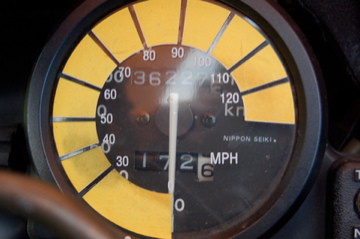The image showcases a speedometer with distinct yellow bars indicating the speed, currently registering at zero. The accompanying odometer shows a mileage reading of 1,726 miles, suggesting minimal usage. The sleek design and clear display offer a precise and user-friendly interface for monitoring the vehicle's speed and distance traveled. The close-up view emphasizes the detailed craftsmanship and easily readable metrics, making it a crucial component of the vehicle's dashboard.